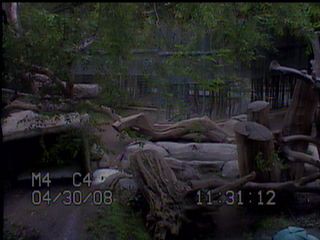The image is a small, grainy still frame, likely from old security camera footage dated April 30th, 2008 at 11:31:12. The scene appears to be set in an outdoor environment with a lot of vegetation, resembling a zoo enclosure. In the background, beyond a wooden fence and scattered logs, boulders, and overgrown roots, you can faintly make out trees and potentially a house hidden behind them. There is a dirt floor with patches of green moss or grass. The left bottom corner of the image has a timestamp and other markings: "M4 C4 04/30/08". The day seems overcast, adding a darker ambiance to the otherwise naturalistic setting.